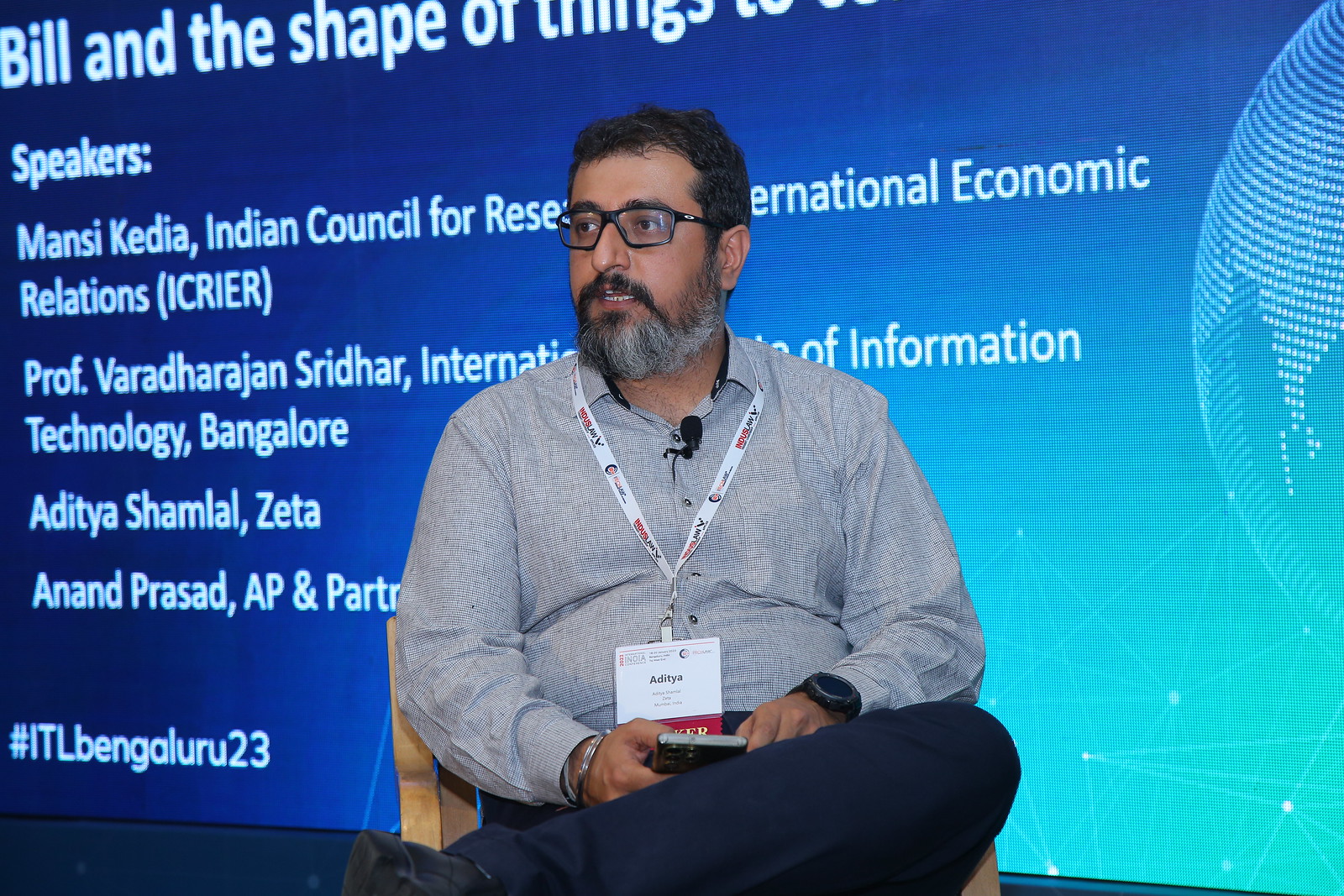In the center of the image sits an older gentleman who appears to be in his 60s. He is seated on a chair, wearing dark-framed glasses, a light blue long-sleeved shirt, and dark blue pants. A ribbon with a name tag hangs around his neck, and he has a prominent black watch on his left wrist. Holding a cell phone in one hand, his legs are crossed and he looks slightly to the left. The gentleman has a distinctive mustache and a beard that is graying, contrasting against his dark hair. 

Behind him, a large screen displays a PowerPoint presentation with a gradient background shifting from dark blue to turquoise. The screen shows a stylized image of a globe on the right, likely representing Asia with India visible. The text reads, "Bill and the Shape of Things," followed by a list of speakers including "Mancy Keita, Indian Council for the Research and International Economic Relations, Professor Vered Harajan Sridhar, Aditya Shambhal, and Arun Prasad." Additional text and a hashtag are partially obscured by the man's head, suggesting that he might be one of the speakers at this indoor event. The overall color scheme of the scene incorporates shades of blue, white, gray, red, tan, and light brown.